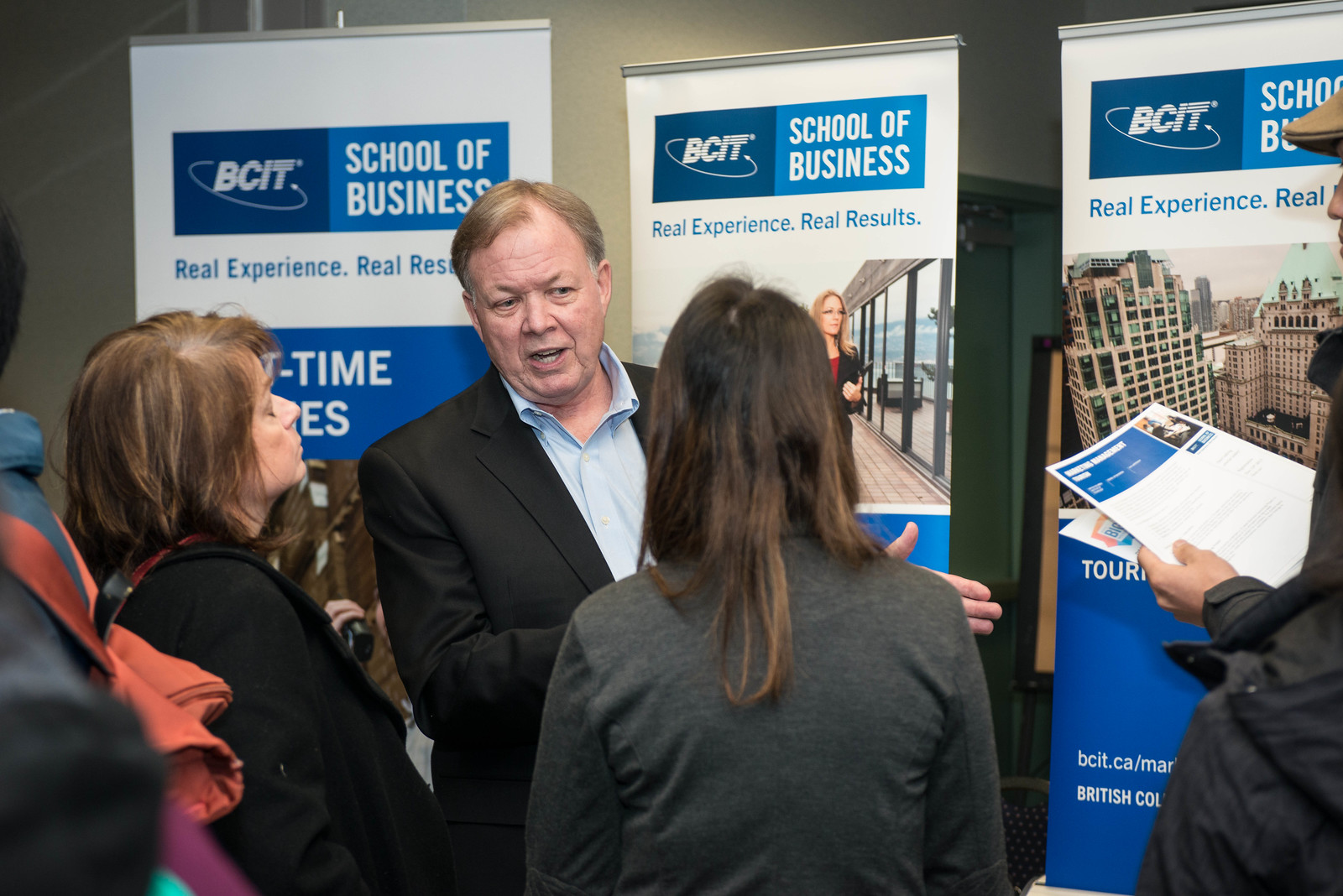In the image, a middle-aged man, appearing to be in his 50s with balding brownish-gray hair, is speaking to a small group of attentive individuals at what seems to be a conference, possibly related to business or education. He is dressed in a black suit jacket paired with a light blue button-up shirt, open at the collar without a tie, and gestures with his hands as he speaks. Behind him, there are three large, floor-length banners, each with a blue logo at the top that reads "BCIT School of Business" alongside the tagline "Real Experience Real Results." The designs on these banners vary slightly: the middle one features an image of a young woman in a business suit standing by glass doors, while the banner on the right displays a high-angle shot of skyscrapers or tall office buildings. The banner on the left is slightly obscured by the people in front of it, making its design harder to discern. The audience, which includes a woman in her early 40s and others who are mostly holding handouts or advertisements, listen intently to the speaker, who could possibly be a professor at the BCIT School of Business, given the context.